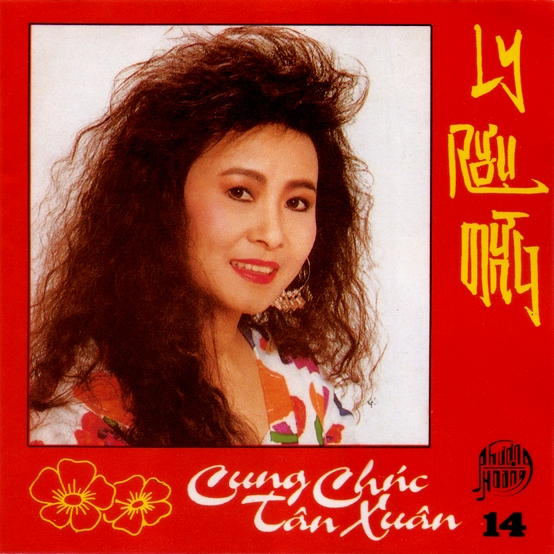This album cover features a predominantly red background with a photograph of a middle-aged Asian woman prominently displayed in the center left, occupying the majority of the image. She has big, frizzy, dark brown hair reminiscent of 80s or early 90s styles, and she wears hoop earrings. Her makeup includes red lipstick and black eyeliner, accentuating her brown eyes. The woman is dressed in a colorful floral-print top, with shades of orange, red, green, and pink. Below her photo, the name "Khang Cheek Tan Zan" or "Sung Chick Tan Xuan" appears in white lettering, flanked by small drawings of yellow daisies on the bottom left. There is a vertical string of yellow Asian text along the right side of the photo, beneath which is a logo or insignia, and the number "14" written in black is visible in the bottom right corner. The background of her photo features a white wall, bordered by the red frame of the cover.